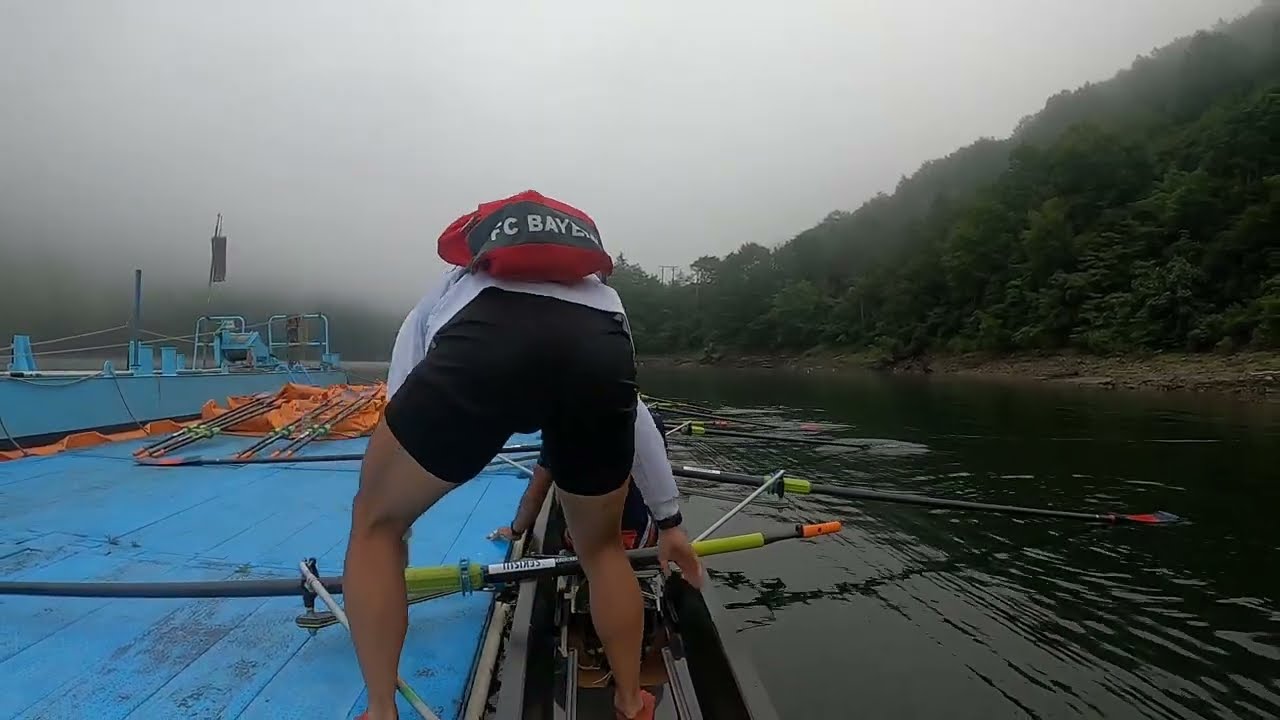The image depicts an outdoor scene with a cloudy, hazy sky in the background. On the left side, mountains loom under the overcast sky, while dense green trees dominate the right. Below these trees, a dirt or sandy bank gently slopes towards the water, which is a dark green, indicating it's likely a river or lake. Central to the image is a person bending over, wearing tight black shorts and a white long-sleeved shirt, identifiable as a male. He has a red and black backpack with "FC Bayern" written on it, slung over his shoulders. The person appears to be interacting with a light blue platform or boat, which has hints of orange and wooden planks. To his right, several rowing oars are visible, suggesting he might be preparing for rowing or some similar activity. The scene is characterized by its somber, potentially rainy atmosphere, lending an overall muted and natural color palette.